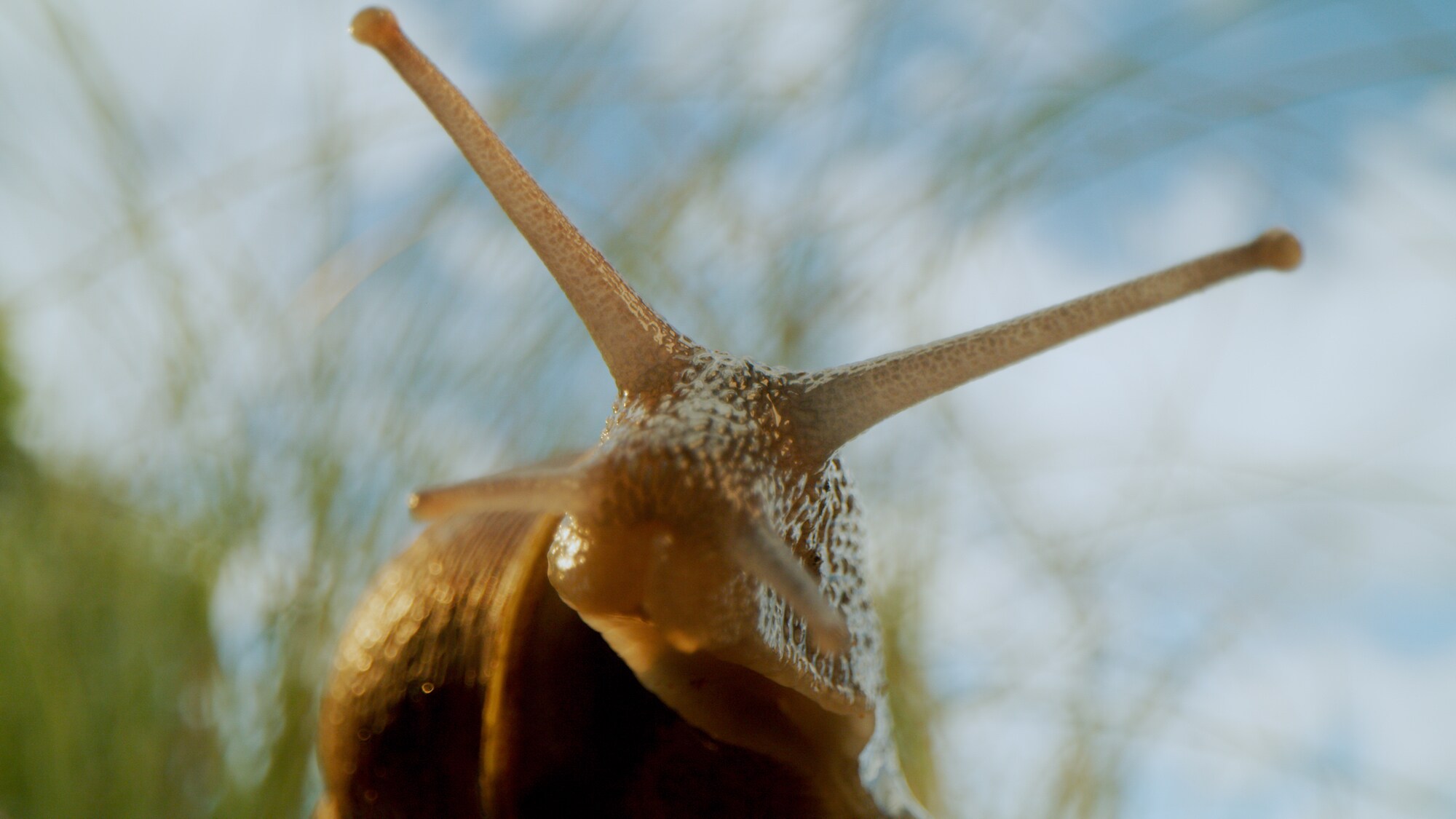The photograph presents an extraordinarily detailed, zoomed-in close-up of a terrestrial snail, set against a backdrop of blurry, tall grasses and a light blue sky with white clouds. The focal point is the snail's head, which highlights its two long, semi-translucent tan-colored tentacles, ending in round bulbous tips, presumably its eye stalks. Below these are two shorter tendrils, also with round bulbous tips. The snail's skin is light brown and appears extremely slimy, adorned with a multitude of small, dimpled bumps. Although the snail's brown shell is visible, it remains out of focus, merging with the indistinct grassy background to keep the observer's attention firmly on the textured, wet surface of the snail itself.